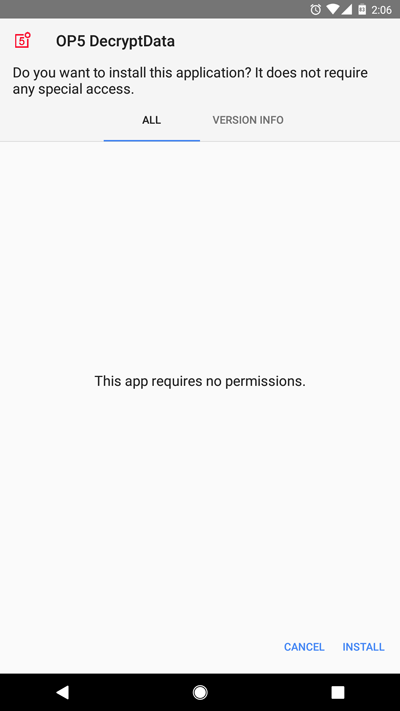This is a detailed screenshot depicting the installation page for an application. At the top-left corner, the application name "OP5 Decrypt Data" is displayed. Adjacent to it, there is a prominently featured red number '5' enclosed within a box. Directly below, a prompt inquires, "Do you want to install this application?" followed by the reassurance, "It does not require any special access." 

Below this information, two tabs are visible: "All" and "Version Info." The "All" tab is highlighted in blue, indicating it is currently selected. Centrally located on the screen is the statement, "This app requires no permissions." 

At the bottom right of the screen, two blue buttons labeled "Cancel" and "Install" are present for user interaction. Beneath these buttons, the device’s navigation bar features three symbols: a triangle for the back button, a circle for the home button, and a square for the menu button, all set against a black background.